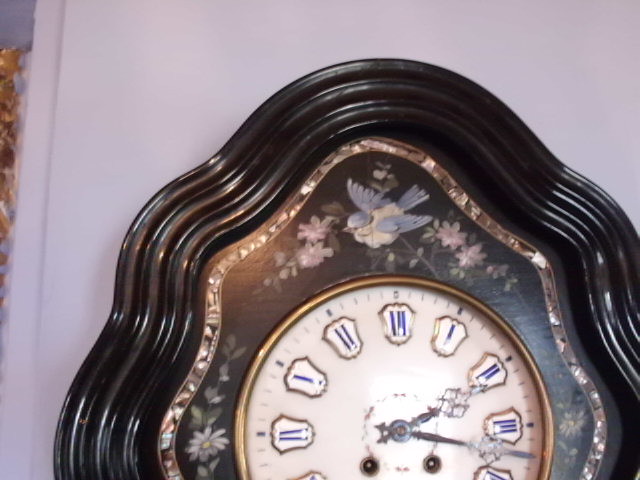This image features an antique-style wall clock mounted on an ivory wall with a subtle pink tint. The clock is distinctly ornate, showcasing a unique oval shape with elegantly undulating wave-like edges. It is encased in a substantial, heavy mahogany wood-like frame that exudes a sense of grandeur. The inlay between the frame and the clock face captures a captivating scene of a bluebird in mid-flight, surrounded by delicate flower petals, with larger flowers accentuating its sides. The clock face is cropped diagonally from 8 o'clock to 4 o'clock, revealing the upper two-thirds of the timepiece. The hands of the clock are intricately designed, and the time displays 2:17. The numbers on the clock are Roman numerals, each set within a gold-edged shield-shaped marking, adding to the clock's antique charm and detailed craftsmanship.